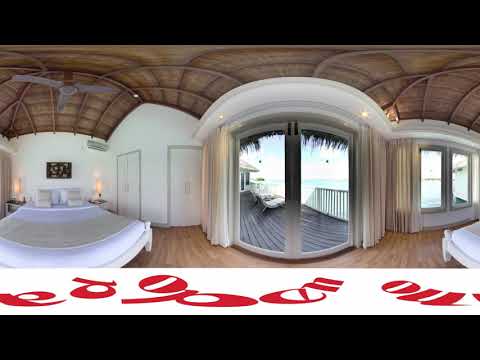The image depicts a panoramic view of a tropical hotel room. On the left, a spacious king-size bed with white sheets and pillows sits against a white wall, adorned with a black painting above it. Next to the bed, there is a bedside table featuring a lamp. The dark wooden ceiling, with its designer pattern and exposed studs, features a three-bladed ceiling fan. Centrally, large sliding glass doors open to a deck furnished with lounge chairs, offering a sunny view of the ocean and what appear to be palm trees, emphasizing the room's tropical setting. The white walls and wooden floor complement the room's airy and warm atmosphere. The right side of the image, due to the fisheye distortion, partially repeats elements from the left, showing the same bed and decor, and revealing additional windows that enhance the room's bright, inviting feel.